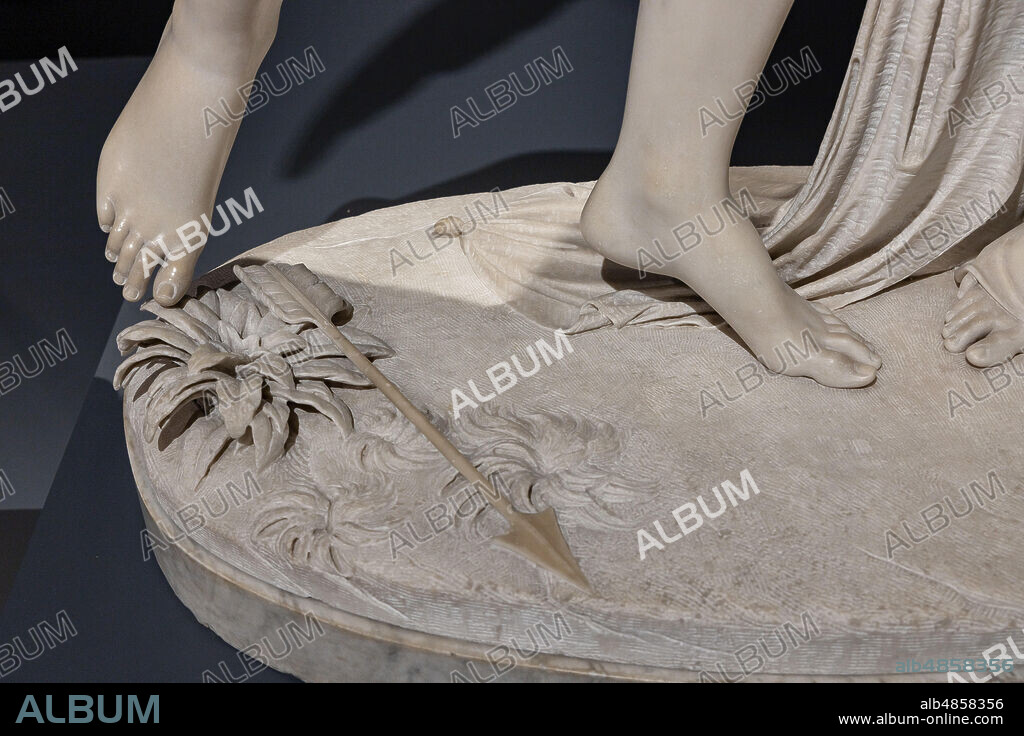The photograph captures a close-up of a marble statue, specifically focusing on the intricate details at the base. The centerpiece features three distinct human feet: one prominently displayed from the front on the left, another viewed from the side, and a third partially visible on the right, seemingly emerging from beneath a draped robe. These feet rest upon a circular stone platform adorned with elaborate carvings of plants and swirling motifs, symbolizing foliage. An arrow, fashioned with an arrowhead reminiscent of Native American design, lies atop the plant carvings. The statue is set against a dark, grayish-blue backdrop, and the word "album" is repeatedly watermarked across the image in varying shades of white and gray. At the bottom, a black line contains the text "ALB4858356" and the website address "www.album-online.com," adding further detail to the composition.